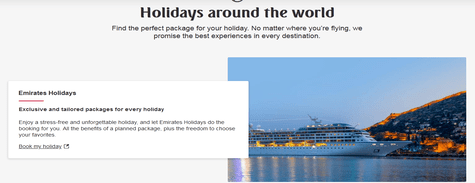This is a cropped screenshot of a section of a travel website, prominently featuring a header that reads "Holidays Around the World" in bold black text. Directly beneath this header is a short description inviting users to "Find the perfect package for your holiday no matter where you're flying. We promise the best experiences in every destination." This suggests a focus on comprehensive travel packages, likely for various types of vacations including cruises. On the bottom-left corner, there is a pop-up labeled "Emirates Holidays" that offers "Exclusive and tailored packages for every holiday. Enjoy a stress-free and unforgettable holiday and let Emirates Holiday do the booking for you. All the benefits of a planned package plus the freedom to choose your favorites." Below this text is a clickable button labeled "Book My Holiday." Adjacent to the pop-up is an image of a large white cruise ship sailing past a strikingly unusual structure with curved architecture and glowing orange lights.